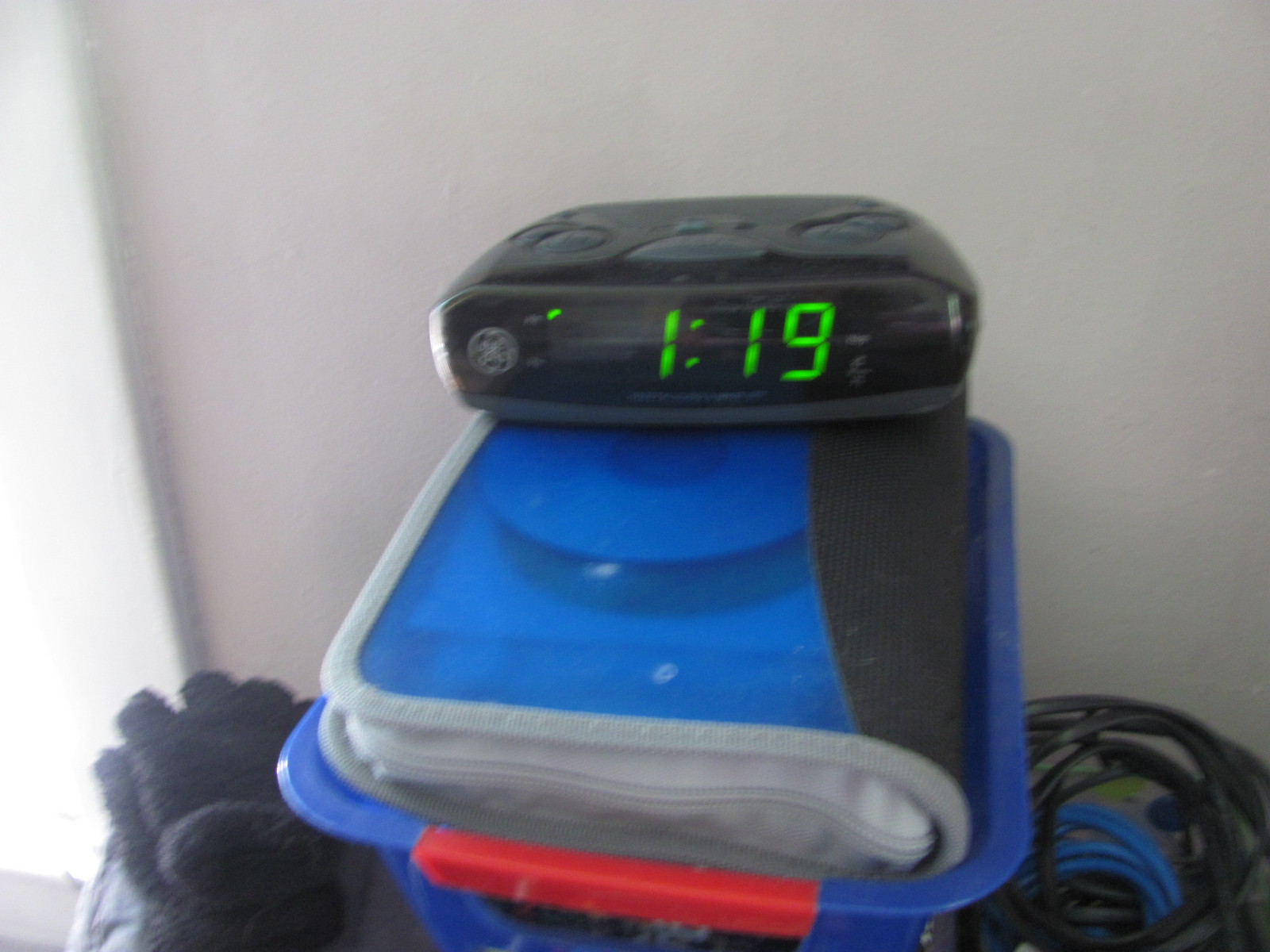This image depicts a low-resolution, blurry photograph showcasing a digital alarm clock positioned on a blue plastic binder, which is presumably a CD or DVD holder. The clock is black and rectangular with a glossy finish and features three large buttons on its top. A circular white GE logo sits on the left side of its face, which displays the time "1:19" in green LED digits. The binder is nested inside a blue plastic tote that has red handles and is part of a cluttered scene with a pile of assorted items around it. To the right of the blue tote, there is a tangle of black extension cords, while to the left, a pair of black gloves and black shoes are partially visible.